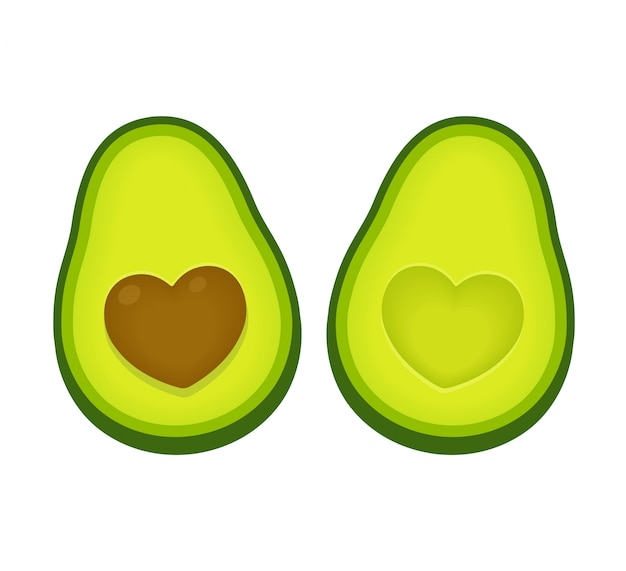This image is a minimalist, cartoon-like drawing of an avocado split in half, with vivid, neon colors. Both halves are set against a plain white background. The left half features a heart-shaped pit in the center, detailed with a brownish hue, resembling a chocolate heart. The colors of the avocado transition from a dark green outer skin, to a lighter green ring just inside, and then an even lighter green towards the center. The right half shows the corresponding indentation where the heart-shaped pit would fit, maintaining the same color gradient from dark green to light green. The halves are mirror images of each other, showcasing the whimsical and vibrant nature of this animated depiction.